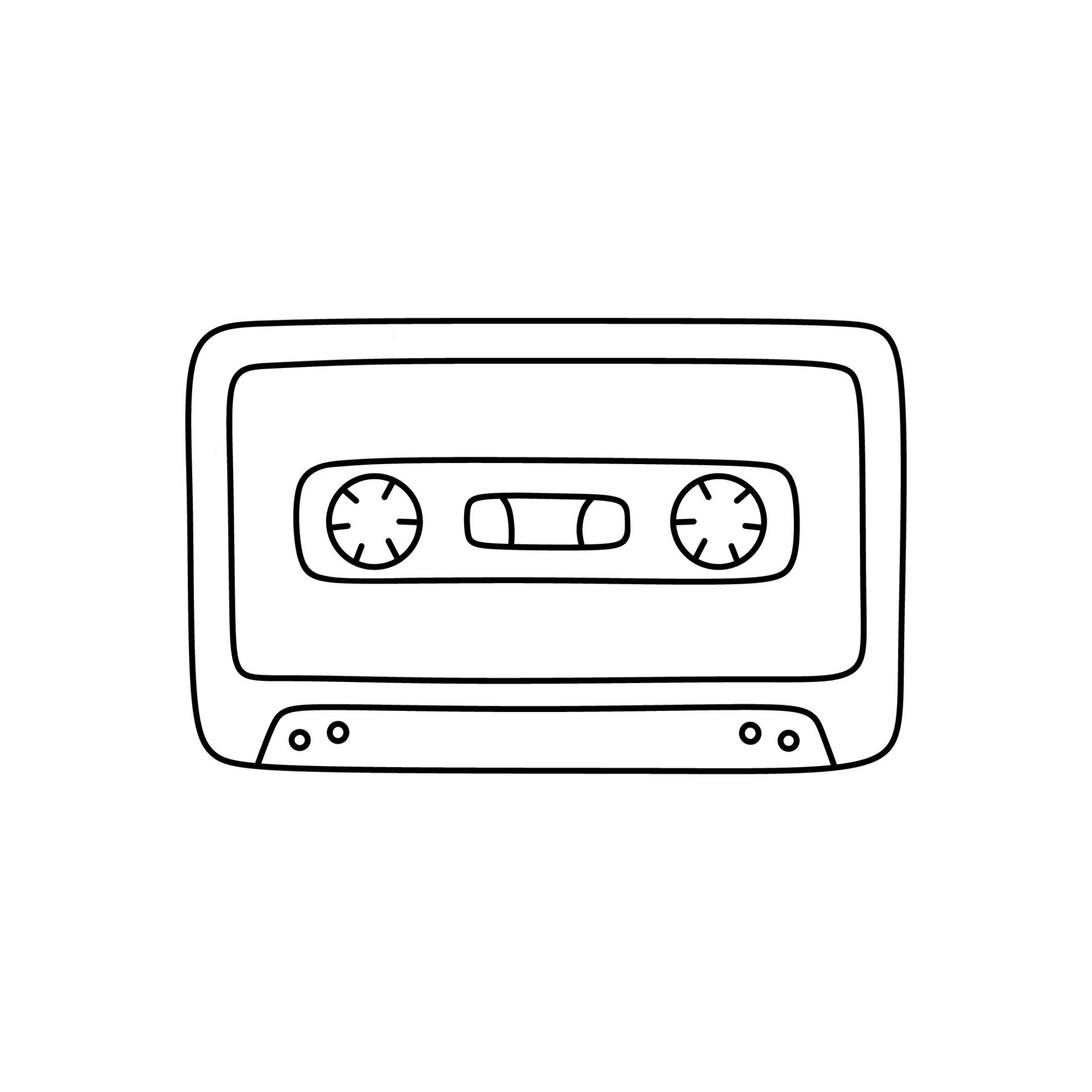The image is a simple black-and-white line drawing of a classic rectangular cassette tape, with the top and bottom edges being twice as long as the left and right sides. Each corner of the tape is rounded, giving it a softer appearance. The tape features an outer rectangle that frames the cassette, within which a narrower inner rectangle represents the label area. Inside this inner rectangle, there is another even thinner, rounded rectangle containing two circles on either side and a smaller rectangle in the center. These circles, complete with small black lines to indicate notches, depict the round wheels where the tape would be threaded into a cassette player. The central smaller rectangle represents the reel tape of the cassette, with curved black lines drawn to illustrate the tape itself. Additional details include four small holes slanted inward located near the bottom left and right sides of the outer rectangle. The background of the image is completely white, enhancing the prominence of the black lines defining the cassette tape's features.